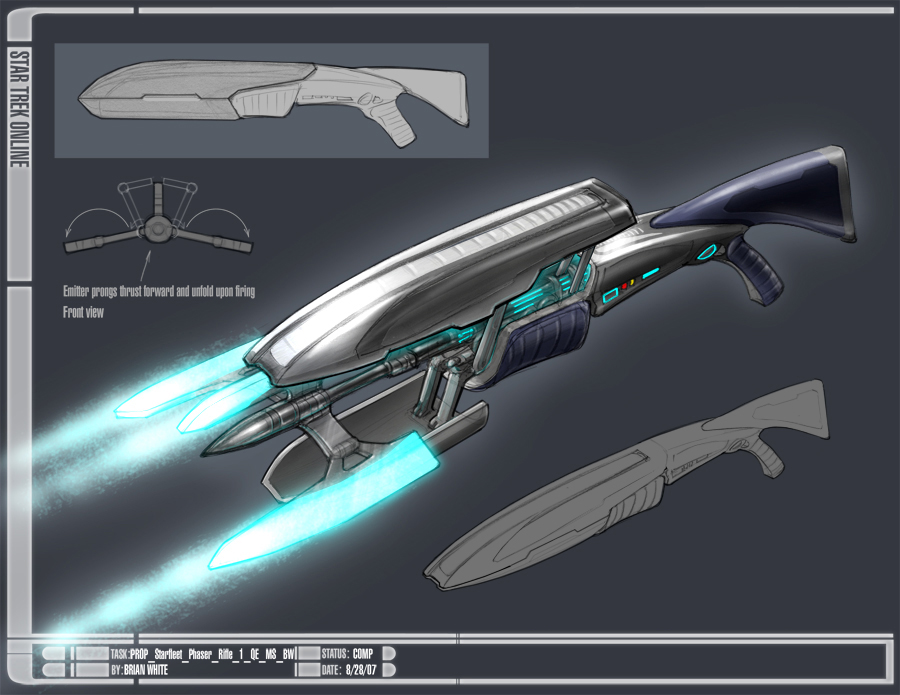The image presents a detailed graphic concept of an imaginary weapon from the Star Trek universe, displayed against a black background with a grey border framing the top, left side, and bottom. The top-left corner features text that reads "Star Trek Online," indicating its association with the game. The central focus of the graphic is a sci-fi phaser rifle, dark grey in color, equipped with a stock, handle, and a barrel on top that emits a blue light, likely representing the phaser beam. Alongside the barrel, blue-lighted prongs extend outward. Below and to the right is a simpler grey drawing of the rifle, shown without any accessories, suggesting an unfinished prototype. Above this, another inset shows a detailed side view of the rifle, with text explaining that "Emitter prongs thrust forward and unfold upon firing, front view." At the bottom of the image, a banner states "Task Prop Starfleet Phaser Rifle 1 QEMSBW" followed by "by Brian White, Status COMP Date 8-28-07," crediting the designer and providing a completion status and date.